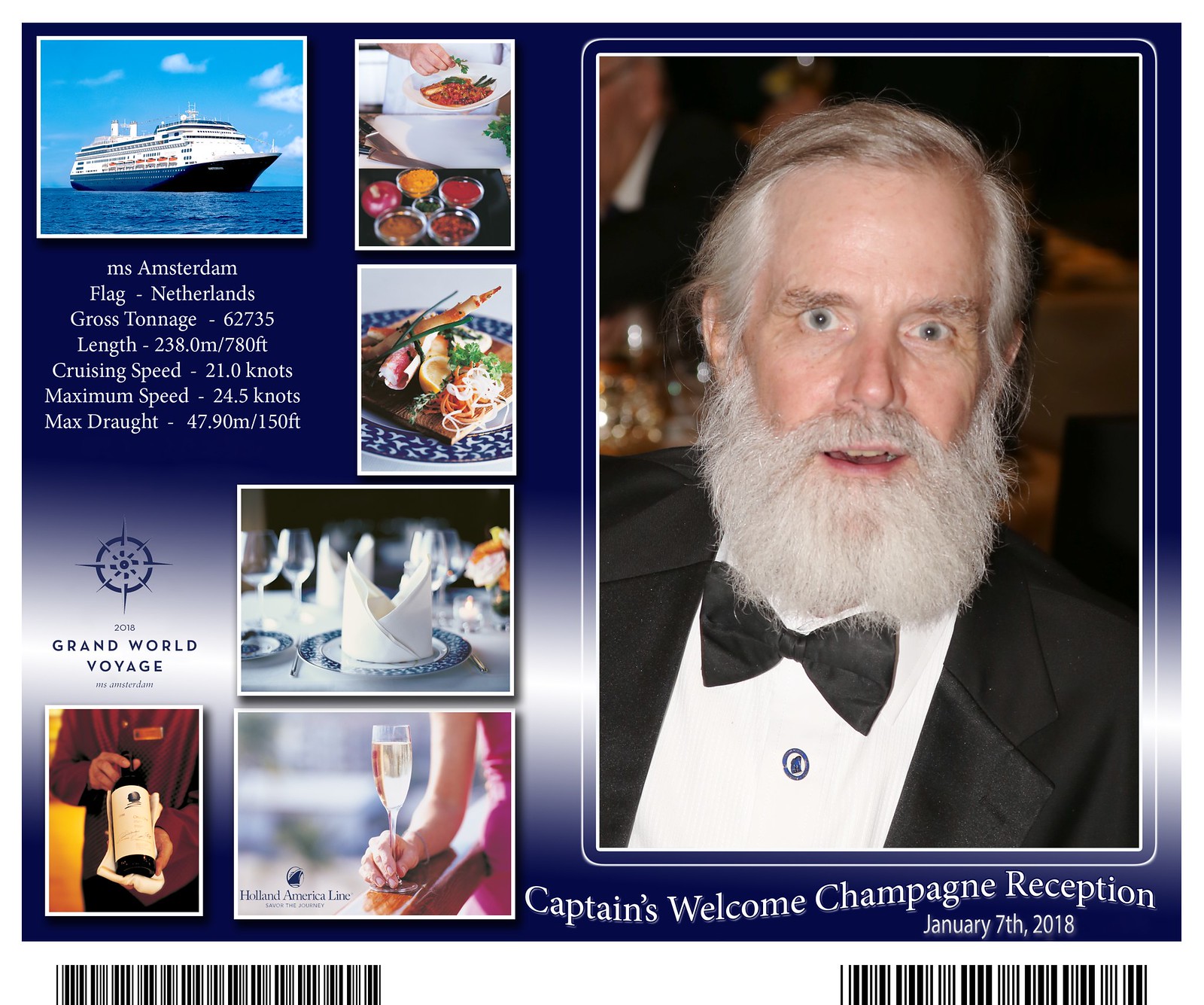The image appears to be a detailed promotional flyer for a Captain's Welcome Champagne Reception on January 7, 2018, for the MS Amsterdam cruise ship. On the right side, there is a photograph of an elderly white man, likely the captain, dressed in a suit and looking directly at the camera. To the left, there are various images including a picture of the MS Amsterdam ship, a dish of spaghetti, an unidentified object beneath it, silverware, a champagne bottle, and a woman holding a champagne flute. The background of the flyer includes informational text about the MS Amsterdam: its flag is from the Netherlands, it has a gross tonnage of 62,735, a length of 238 meters, a cruising speed of 21 knots, a maximum speed of 24.5 knots, and a maximum draft of 47.9 meters. The color scheme of the flyer predominantly features white, black, gray, tan, blue, pink, orange, and yellow. The overall design of the flyer suggests it's an elegant invitation to the reception event hosted on the cruise ship.